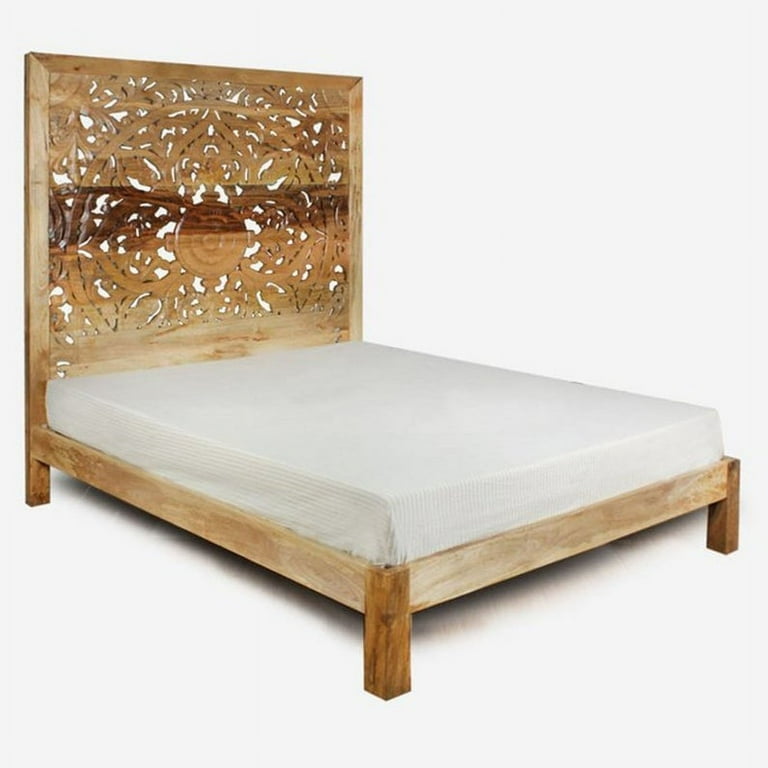This image appears to be an advertisement for a bed, showcasing a minimalist yet striking design. The bed prominently features a white mattress, which has a corduroy-like texture and appears to be covered with a white sheet. The mattress rests on a wooden bed frame, which is constructed from natural, light-colored wood with visible dark grains. The base of the bed is supported by four legs, although only three are visible in the image due to the perspective.

Dominating the background of the image is a massive wooden headboard, intricately designed and almost the same size as the bed itself. The headboard is a work of art, with numerous geometric cut-out patterns including a central circle that radiates out into various shapes, creating a captivating and open design through which the white background shows. The room is stark and devoid of any other elements, emphasizing the bed as the focal point against a clean, all-white backdrop.